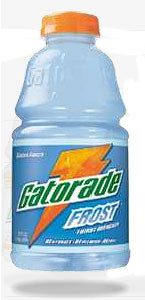Product Photograph of Gatorade Frost: This detailed image showcases a 28-ounce Gatorade Frost bottle, prominently centered and facing front to display its label clearly. The bottle is crafted from clear plastic, allowing the frosty light blue color of the electrolyte beverage to be visible. It features an orange plastic cap. The label, set against a white background, reads "Gatorade" in a green font with an orange lightning bolt cutting through the brand name. Below, the word "Frost" is styled in light blue with subtle white gradients at the edges of each letter, emphasizing the frosty theme. This product is specifically designed for hydration and to replenish fluids when dehydrated. The overall presentation of the photograph mimics that of an online shopping advertisement, focusing on clarity and detail.